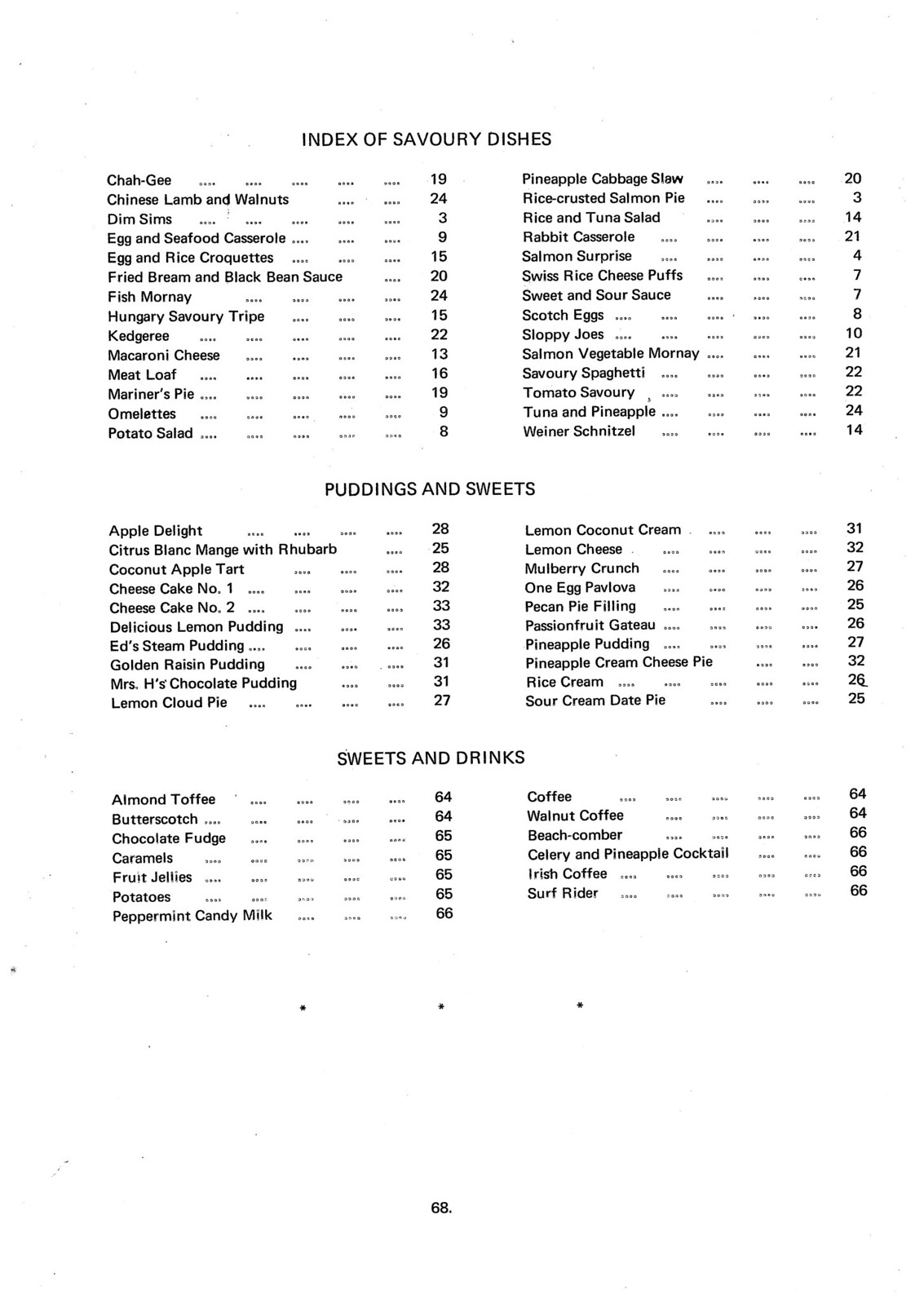This is a detailed, cleaned-up caption for a given image of a list with a clear layout:

---

This image is either a screenshot or a scan of a meticulously organized list, printed in black font on a white background. The list is titled "Index of Savory Dishes," acting as the main header. Below the header, the content is categorized into two columns.

On the left column, the entries are as follows:
- Cha Gee, page 19
- Chinese Lamb and Walnuts, page 24
- Dim Sims, page 3
- Egg and Seafood Casserole, page 9
- Egg and Rice Croquettes, page 15
- Fried Bream and Black Bean Sauce, page 20
- Fish Mornay, page 24
- Hungry Savory Tripe, page 15
- Ked Geary, page 22
- Macaroni and Cheese, page 13
- Meatloaf, page 16
- Mariner's Pie, page 19
- Omelets, page 9
- Potato Salad, page 8

The right column contains the following items:
- Pineapple Cabbage Slaw, page 20
- Rice Crusted Salmon Pie, page 3
- Rice and Tuna Salad, page 14
- Rabbit Casserole, page 21
- Salmon Surprise, page 4
- Swiss Rice Cheese Puffs, page 7
- Sweet and Sour Sauce, page 7
- Scotch Eggs, page 8
- Sloppy Joes, page 10
- Salmon Vegetable Mornay, page 21
- Savory Spaghetti, page 22
- Tuna and Pineapple, page 24
- Wiener Schnitzel, page 14

Following this extensive index of savory dishes, the categories "Puddings and Sweets" and "Sweets and Drinks" also make an appearance, each with their respective lists laid out underneath. Finally, at the very bottom of the page, the number "68" is prominently displayed, most likely denoting the total page count of the document.

---